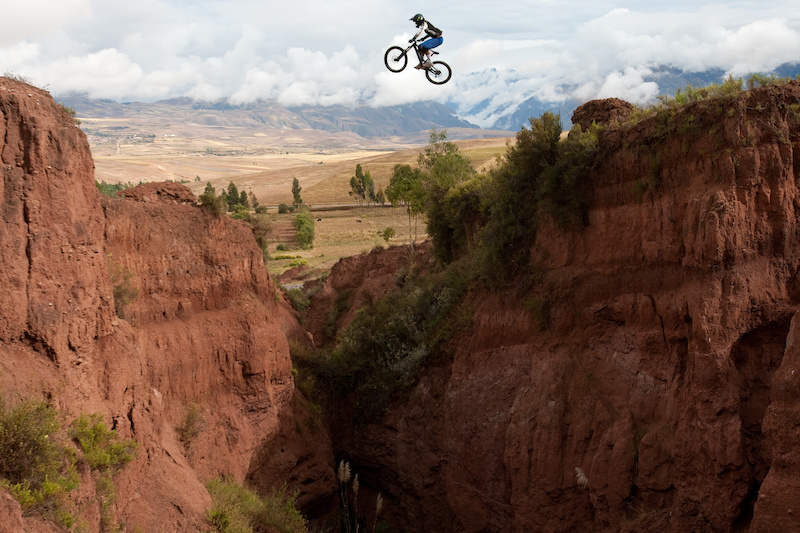This captivating image showcases a dramatic scene of a biker mid-jump between two large, steep cliffs resembling the beige tones of the Grand Canyon. The cliffs are accented by olive green bushes and pampa grass, with lush vegetation more densely packed on the right side. The biker, wearing a black helmet, blue shorts, a white shirt, and possibly a black backpack, is airborne, seemingly attempting to bridge the gap from the left cliff to the right. His black bicycle is tilted with the front wheel higher than the back, indicating an upward trajectory. The background features a barren, brown-yellow landscape dotted with sporadic green trees that roll into distant foothills shrouded in white clouds and fog. The dramatic setting and the daring stunt evoke a sense of adventure reminiscent of Evel Knievel.